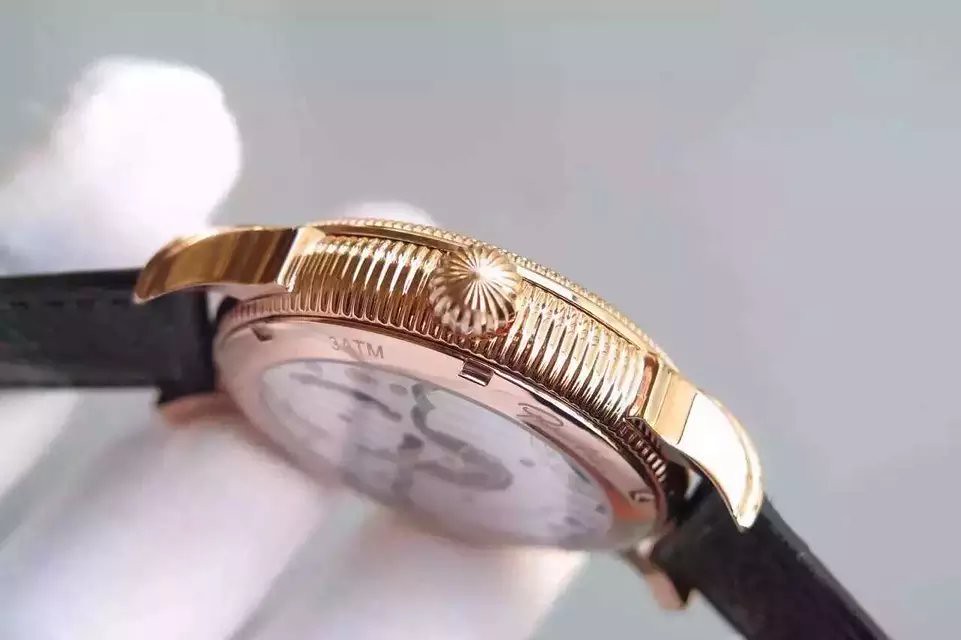The image showcases a detailed side view of a wristwatch, focusing on its bezel. The bezel, which is either gold-plated or made of actual gold, prominently features the knob used for adjusting the time, date, or winding the watch if it is a mechanical model. Black straps extend from the bezel, secured by two clasps, adding a contrasting elegance to the gold. Though the face of the watch is partially obscured from this angle, it is discernible that the watch has a white face. The intricate interplay of the gold bezel, black wristbands, and white face encapsulates a timeless, sophisticated design.